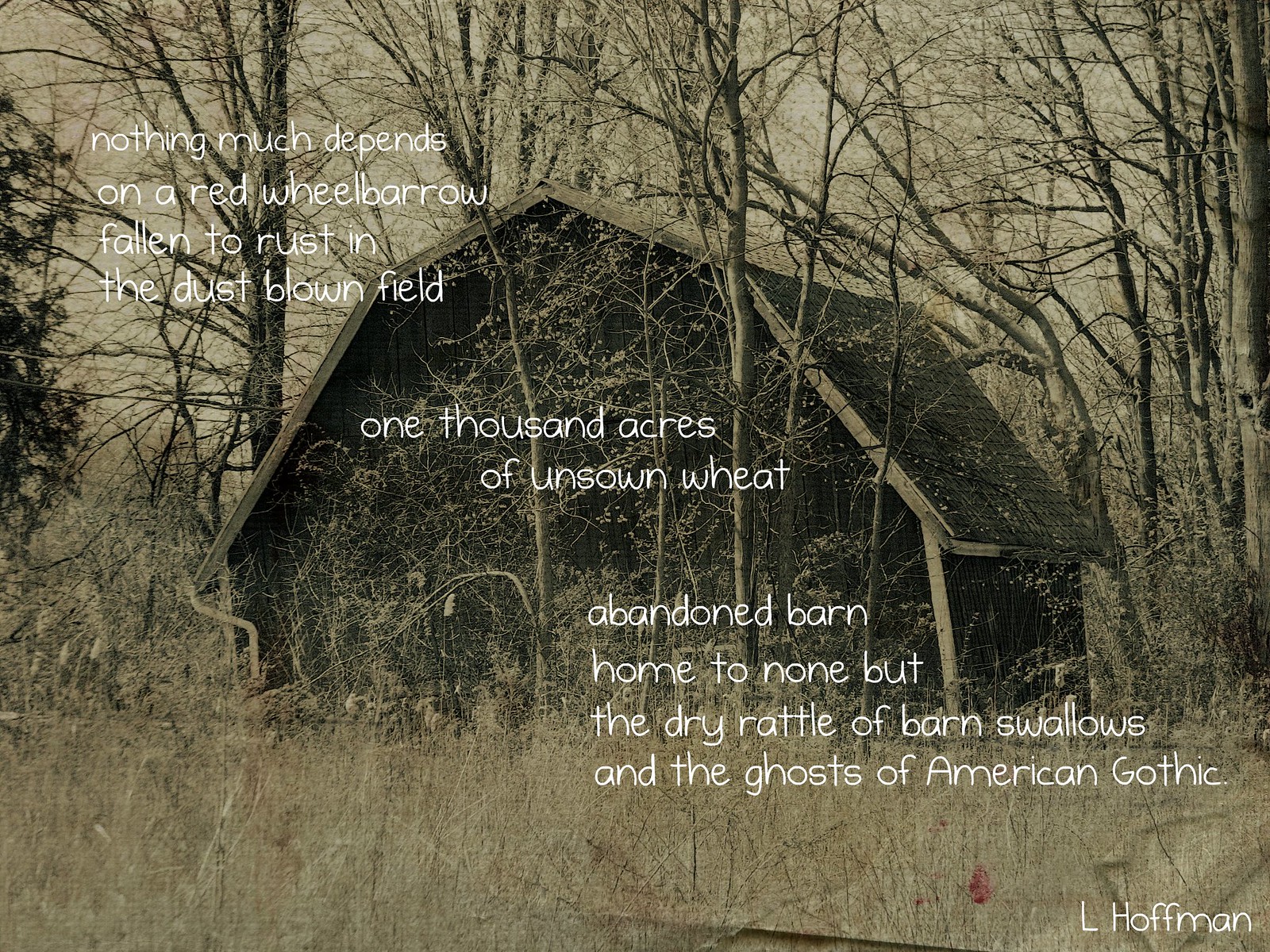The image features an inspirational quote superimposed on a black-and-white photograph of an overgrown, abandoned barn. The barn, with its four-sided roof and white trim, lists to the side amidst a setting dominated by multiple leafless trees, giving it an eerie, desolate appearance. The surrounding area is a dust-blown field with tall, yellow grass and mentions of an expanse of 1,000 acres of unsewn wheat. The poignant quote reads, "Nothing much depends on a red wheelbarrow fallen to rust in the dust-blown field. One thousand acres of unsewn wheat, abandoned barn, home to none but the dry rattle of barn swallows and the ghosts of American Gothic." This text is presented in white font, with the name L. Hoffman appearing at the bottom right. The entire scene has a vintage, timeless quality, enhancing the sense of abandonment and nostalgia.